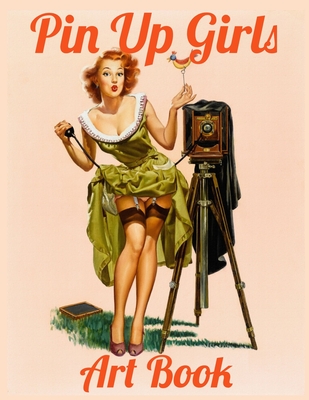The cover of the art book, styled reminiscent of the 1950s or 60s, features a striking pin-up girl design against a light pink or peach background. At the top of the cover, bold red or orange script reads "Pinup Girls," while the bottom of the cover features the matching text "Art Book." Dominating the center is a vividly detailed illustration of a woman with vibrant red hair, styled in loose waves. She is dressed in a low-cut, flowy green dress adorned with white frills at the shoulders, pulling up her skirt to reveal black lingerie-style stockings held up by a garter belt and white panties peeking from underneath. She stands in a flirtatious pose, with knees together and high-heeled shoes accentuating her legs. Her lips are pursed in a playful kiss, accentuated with red lipstick. Beside her is an antique camera mounted on a tripod, complete with a black hood draped over it and a cord that the woman holds, lifting her skirt in the process. The entire scene evokes a classic and nostalgic feel, perfectly capturing the essence of vintage pin-up art.